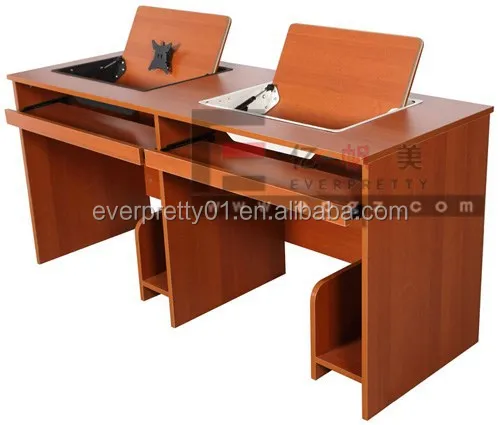The image features a detailed, rectangular desk with a rich cherry wood finish, showcasing various shades of brown and darker brown throughout the wood grain. The desk is divided into two compartments side by side, with distinct upper and lower sections. The top shelf is a connected piece, hosting areas designated for placing laptops or computer monitors. Each side of the desk includes a keyboard holder embedded within cutout sections and individual built-in shelves located on the bottom right-hand side of each compartment.

Additionally, the desk is equipped with several wooden drawers that are partially pulled out, separated by vertical wooden slabs which segment the middle from the left and the right sides. These slabs also feature inward-turning wooden panels suitable for propping up an iPad or tablet, facilitating an upright workspace for digital tasks. Spanning across the middle of the image is a watermark with the text "everpretty01.en.alibaba.com," accompanied by another watermark with Chinese characters conveying the same message.